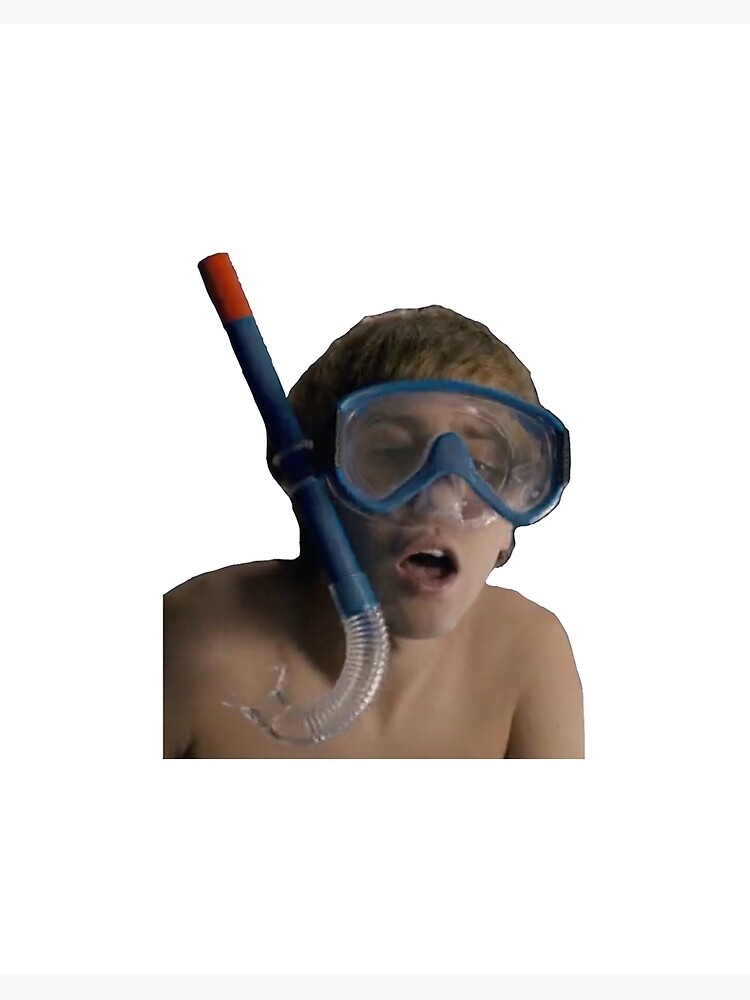This is a photo of a young white boy, likely between the ages of 11 and 15, set against a stark white background, which suggests the image has been cut out, possibly with crude Photoshop work. The boy has short, light brown hair and is bare-chested, with only the top of his chest, shoulders, and arms visible. He is equipped with snorkel gear: goggles perched on his forehead and a snorkel hanging from the goggles with a clear mouthpiece, a dark blue-teal body, and a red tip. His mouth is open, revealing his front teeth, and his eyes appear to be closed or looking downward, giving an impression of either distress or deep breath preparation. The white background and the ragged outline further convey that the image was extracted from its original context.